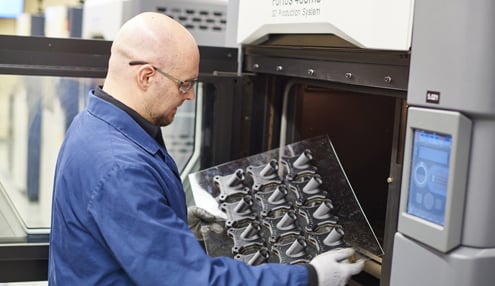This photorealistic image captures a detailed scene of a middle-aged, bald man with a short-trimmed goatee and safety glasses, dressed in blue overalls and gray gloves. He is holding a large sheet of glass or plexiglass with a series of small metal objects bolted onto it, appearing to either load or unload it from a machine. The man, standing on the left half of the image and looking to the right, is positioned in front of a sizable, gray machine with a black oven-like interior. The door of the machine, which is framed in black metal and has a clear glass insert, is open behind him. To the right of the machine's opening, there is a blue light-up control panel. The man is visible from his head down to his elbow, highlighting his focused profile as he interacts with the equipment.